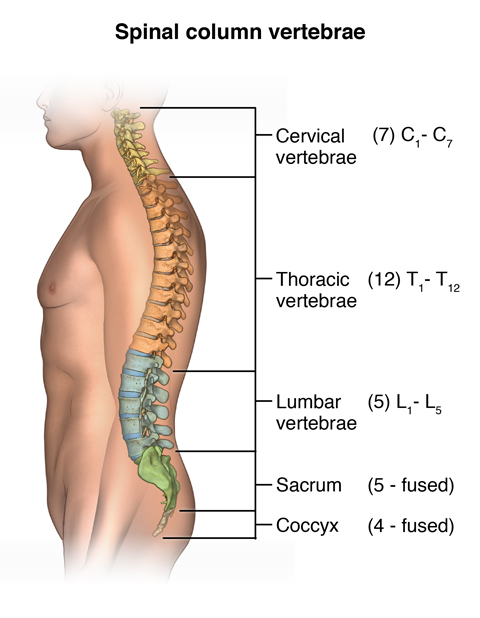The image depicts a detailed side view of a human body, with a focus on the spinal column vertebrae. At the top center of the illustration, it reads "Spinal Column Vertebrae." The outline of the human figure acts as a backdrop, with the internal vertebrae prominently highlighted and color-coded to distinguish different parts of the spine. 

The top section is labeled as "Cervical Vertebrae" and consists of 7 vertebrae (C1 to C7). Moving down, the next section is the "Thoracic Vertebrae" which contains 12 vertebrae (T1 to T12). Below the thoracic section, the "Lumbar Vertebrae" are highlighted, consisting of 5 vertebrae (L1 to L5). Further down, the "Sacrum" is illustrated as a section of 5 vertebrae fused together. The smallest part at the base is the "Coccyx," which comprises 4 fused vertebrae.

The spinal sections are color-coded for clarity: the cervical vertebrae are yellow, the thoracic vertebrae are tangerine, the lumbar vertebrae are blue, the sacrum is green, and the coccyx is pink. Additional lines and labels point to each segment, providing a clear, organized chart that illustrates the structure and division of the spinal column.